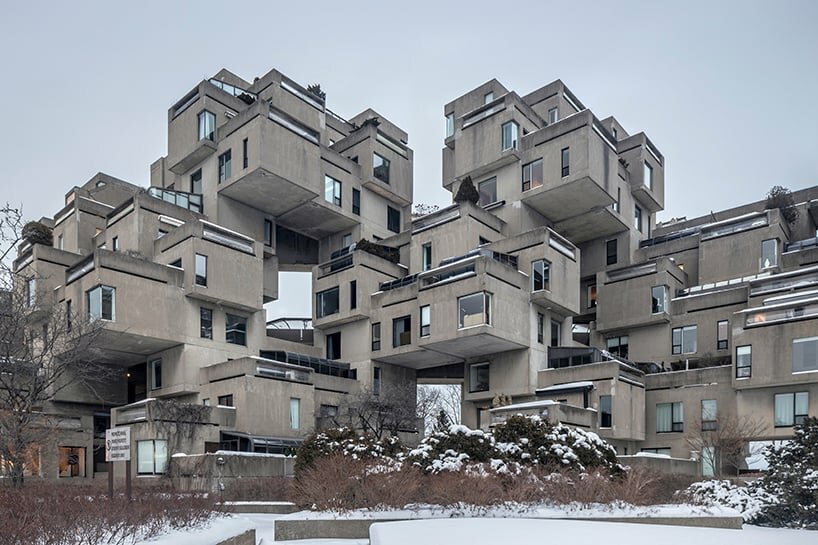The image depicts a large grayish building made of cement with a distinctive architectural design characterized by a series of interconnected, floating blocks. These blocks, resembling square boxes, are cleverly cantilevered, creating overhanging sections that appear to float or hang off the sides. The building displays numerous flat-topped, windowed sections, some extending without direct support beneath. The structure, which could be either a business complex or housing units, stands amidst a snowy landscape with snow-covered bushes. In the background, the sky is gray and cloudy, adding to the overall drab atmosphere. A blurry sign is visible on the left side of the image, though its text is unreadable. The unique design includes open holes through the building, offering intriguing views through its various angles and connections.